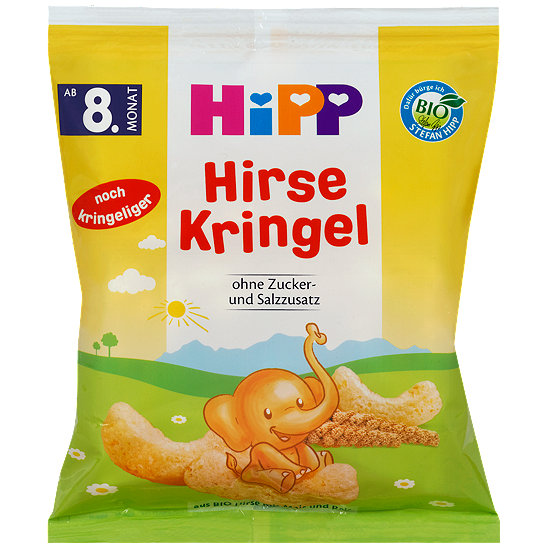The image depicts a vividly colored package of puffed snacks designed for young children, prominently displaying the brand name "HIPP" in playful, multicolored letters (H in pink, I in blue with a heart instead of the dot, and both P's with heart cutouts in orange and purple). The package features a sealed plastic bag with a narrow white strip at the top and a dominant yellow background that transitions to green at the bottom, representing grass and hills. An orange elephant with a joyful, smiling expression sits atop a curl-shaped cheesy puff, surrounded by a whimsical scene with a yellow sky, green trees, and flowers. Below the brand name "HIPP," the words "Hirsch Kringle" are written in red font, followed by the German phrase "OHNE Zucker-Und-SALZZUSATZ" in black, indicating it is free of added sugar and salt. In the upper right corner, a blue seal with "BIO" in green letters and a leaf icon suggests the snack is organic. Additionally, the upper left corner has a purple background with "8+ Mon" likely indicating the snack is suitable for children 8 months and older.